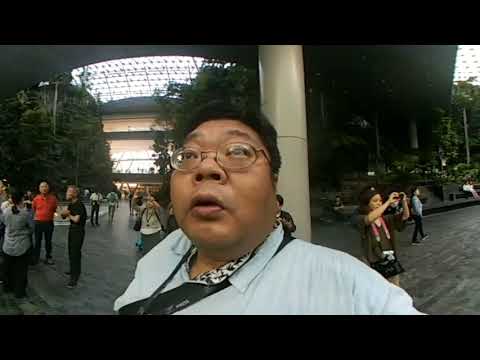A close-up image features a man with a round face, short black hair, and glasses, looking upward with a somewhat surprised expression. He is wearing a light blue shirt with a white collar and a black lanyard around his neck, possibly attached to a camera or bag, which hangs over his chest. The background is slightly blurry, populated with several people standing around, including a person on the right who is taking a picture and a small group of three individuals huddled together on the left. A white pillar stands directly behind the main subject, with some greenery visible on the right side. Additionally, there are tall trees and hints of the sky peeking through what appears to be an indoor setting, possibly in a tourist area with framing elements visible at both the top and bottom of the image.